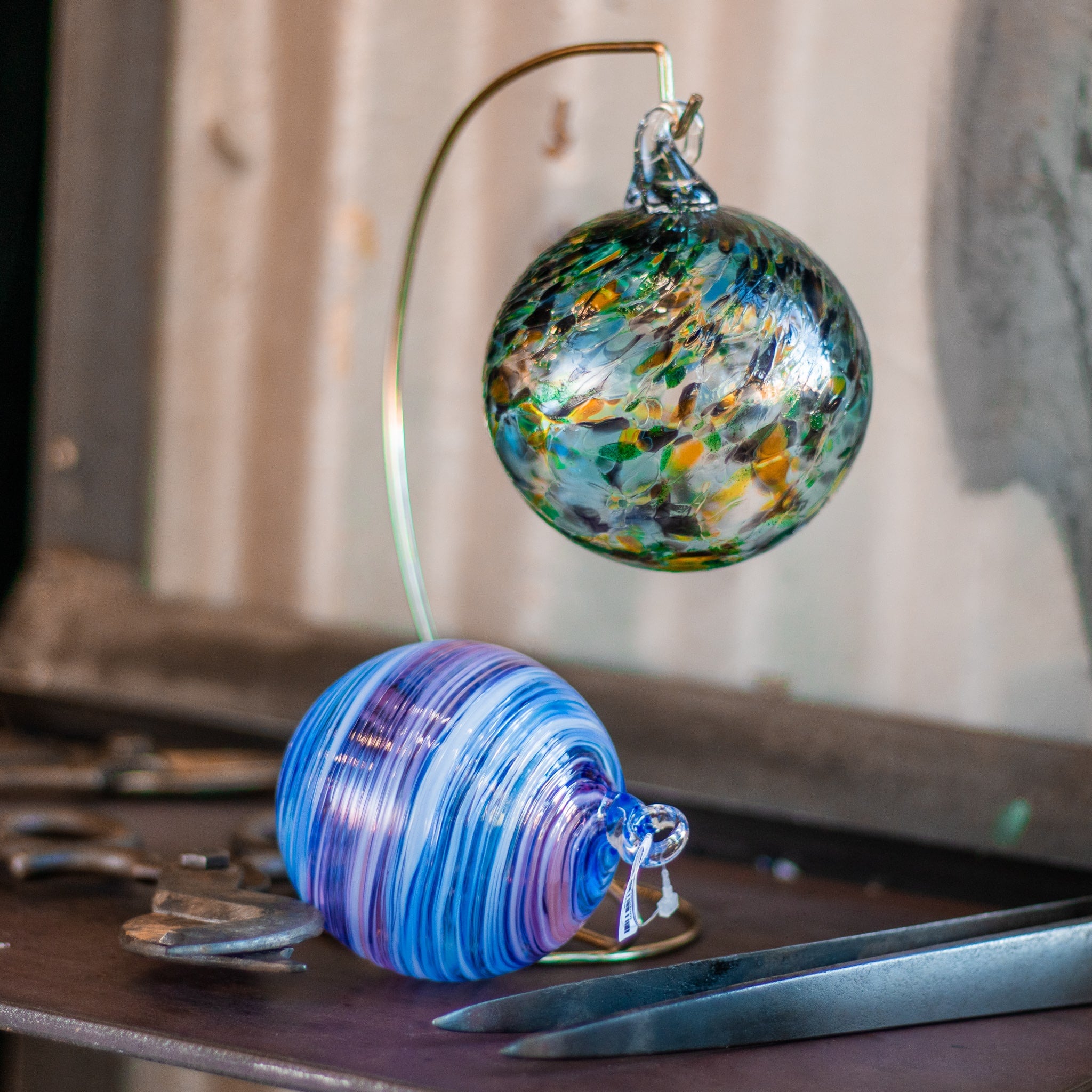The image showcases a detailed close-up of two glass Christmas decorations or baubles displayed on a dark brown, wooden table. The bauble that is hanging from a metal stand features a dazzling array of colors, with blotches of green, yellow, blue, and potentially black, all mixed together in a manner reminiscent of stained glass. Directly beneath this bauble lies another glass ornament, which boasts an intricate swirl pattern in shades of white, light blue, purple, and turquoise—evoking the appearance of ocean waves. This lower bauble still bears a barcode tag, indicating its newness. Accompanying these decorations, the table also holds a pair of silver metal tweezers and what seems to be another scissor-like tool with a wide tip, positioned behind the lower bauble. The background remains blurred and whitish, bringing the vibrant details of the baubles into sharp focus.